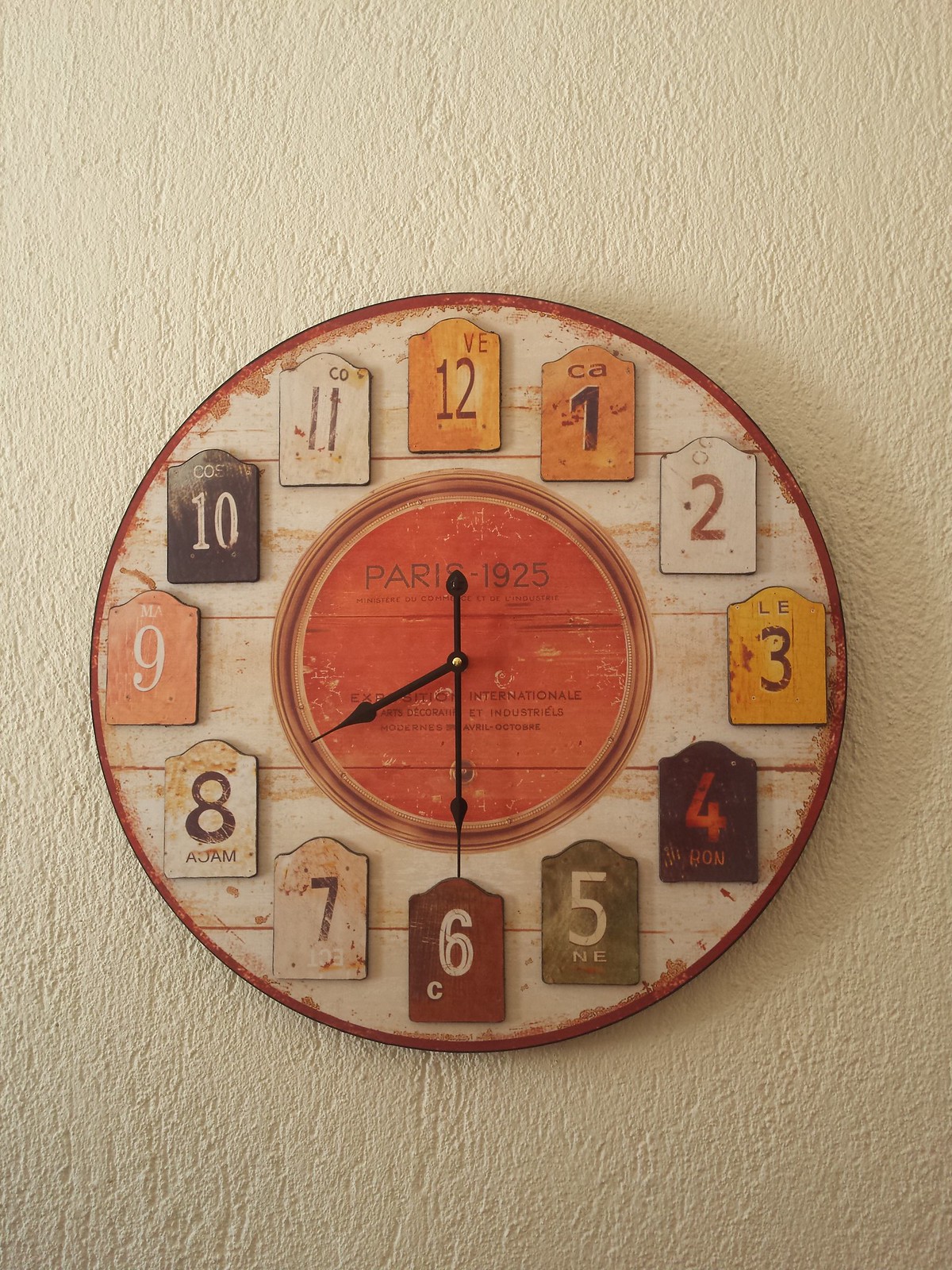This image features an artistic clock mounted on a rough, white-painted cement wall that exhibits numerous indentations, giving it a highly textured and porous appearance. The clock stands out with its vivid orange outer ring, which shares the porous texture of the background. The clock face is intriguingly created from horizontal slats of wood, varying in hues of tan, orange, and brown. The clock hands are positioned at 8:30. Adding to its artistic flair, each hour is marked by a distinctively colored tab with different backgrounds and text colors, making it as much a decorative piece as it is functional.